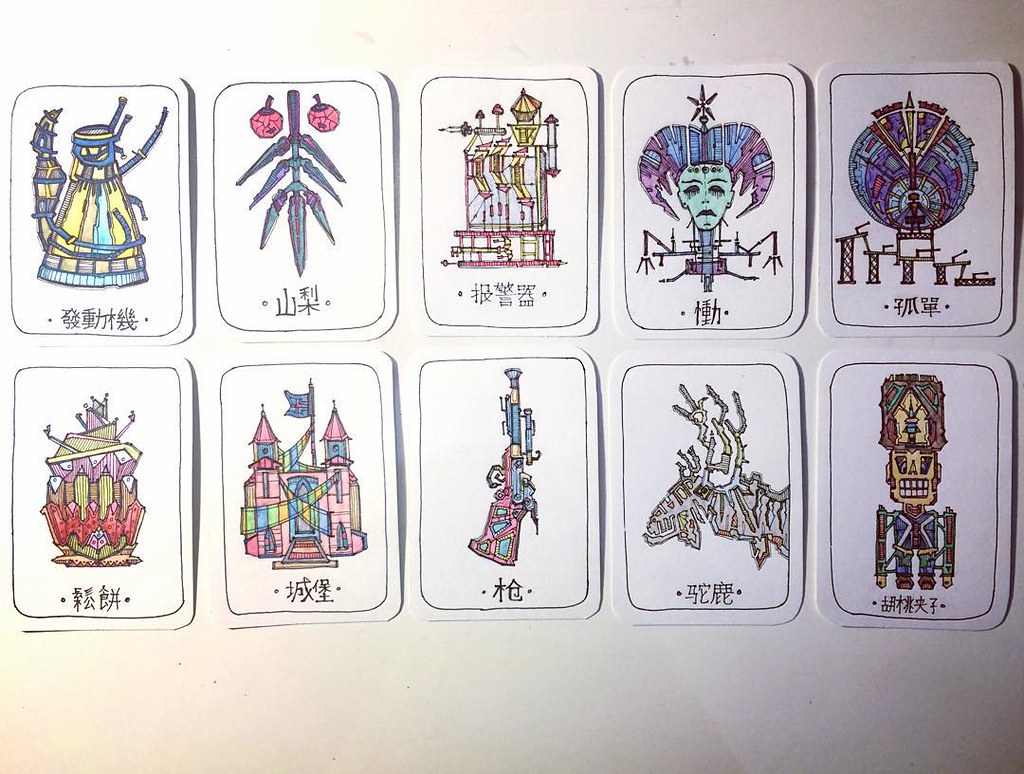This image depicts an intriguing array of ten cards, which initially may appear to resemble tattoo stencils but unfold into a captivating display of unique illustrations and enigmatic text. The cards are arranged in two rows of five, each showcasing diverse and intricate designs accompanied by inscriptions in an unfamiliar script, possibly a language or descriptive terms.

Starting from the top left:
1. The first card features an abstract image, the colors dominated by yellows and blues, vaguely resembling a ship or maritime vessel.
2. The second card portrays a dagger, pointed downward, hinting at its potential symbolic meaning.
3. Moving right, the third card reveals a machine in operation, its purpose and mechanics left to the viewer's imagination.
4. The fourth card displays what seems like a ceremonial mask, evoking the artistic styles of traditional African masks with intricate details and cultural significance.
5. The fifth card on the top row has a futuristic, cylindrical object adorned with mechanical components.

On the bottom row:
1. The card on the extreme left depicts a house, rendered in vibrant color choices.
2. Adjacent to it, a card illustrates a castle, accented with a whimsical palette of pinks, blues, and yellows.
3. The middle card unmistakably features a weapon, possibly a handgun or rifle, with precise detailing.
4. Next, an animalistic figure graces the card, reminiscent of a deer with a pronounced snout, neck, and protruding horns.
5. The final card on the bottom right bears a resemblance to a nutcracker figurine, complete with a tall hat, a face, and a well-defined body structure.

Each card combines artistic creativity with a mysterious narrative, encouraging viewers to delve deeper into its visual elements and speculative meanings.